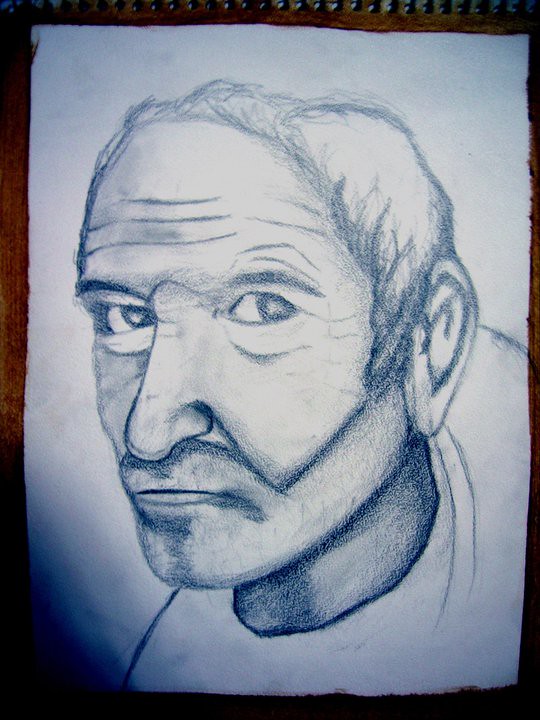A captivating image showcases a portrait framed with a black border, featuring a piece of paper in the center. The focal point of the portrait is a man captured in profile view, looking to the side. He has short hair and notable features, including slightly deformed ears and a forehead marked with three distinct wrinkles, with the longest wrinkle at the bottom.

The individual's eyebrows are carefully detailed, and a prominent line can be seen above the bridge of the nose, providing depth to the facial structure. The nose itself is well-defined with shading that further emphasizes its shape. The lips are pursed, and a prominent cheekbone draws attention to the contour of the face.

Below the face, the neck also displays signs of age with slight wrinkles, and the shirt worn by the individual is depicted with meticulous folds, indicative of fabric texture. The entire piece appears to be skillfully rendered in black ink, lending a dramatic and timeless quality to the portrait.